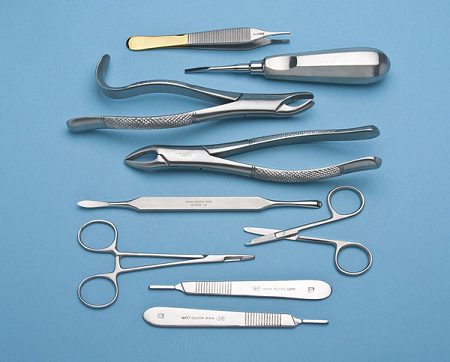The image is a detailed photograph showcasing an assortment of silver tools neatly aligned on a light blue background. At the top, there is a set of tweezers, followed by a tool resembling a screwdriver or an applique tool, possibly for applying small gems. Below that, there is another set of tweezers with a spring-action mechanism for easy opening and closing. The subsequent tool is a pointed object, perhaps used for cleaning under nails. Next, there is a small pair of scissors, likely for fine tasks such as trimming eyebrows, and a larger pair of scissors placed below it. Additionally, there are tools that look like files, useful for refining and cleaning nails. Each tool is meticulously aligned, alternating in direction, adding to the orderly presentation. This collection of tools could be from a medical or dental kit, or possibly for detailed nail care, indicating their versatile uses in professional or personal grooming contexts.